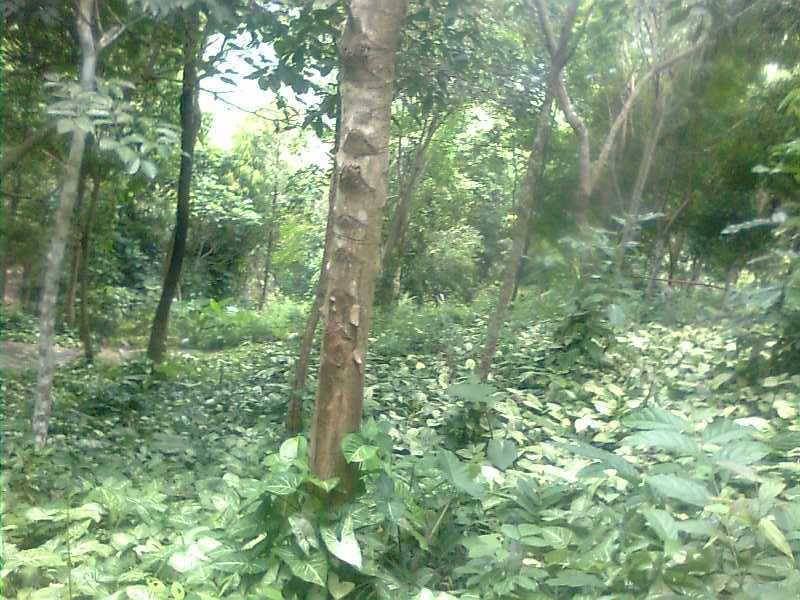The photograph captures a serene outdoor scene in an open woodland or forest on a bright day. The landscape orientation reveals a forest floor blanketed in green ivy, vines, and scattered leaves. Thin, tall trees are dispersed throughout, with their branches and sparse foliage seen primarily in the upper sections of the image. In the background, a dense wall of thick foliage creates a lush, verdant backdrop. A narrow, somewhat indistinct path snakes from the middle left and veers off slightly to the right before disappearing into the greenery. The upper right corner of the image appears blurry, though this blur is not due to motion. A patch of light blue sky peeks through the canopy, adding a hint of brightness to the scene. The image presents a realistic and detailed representation of the forest environment.